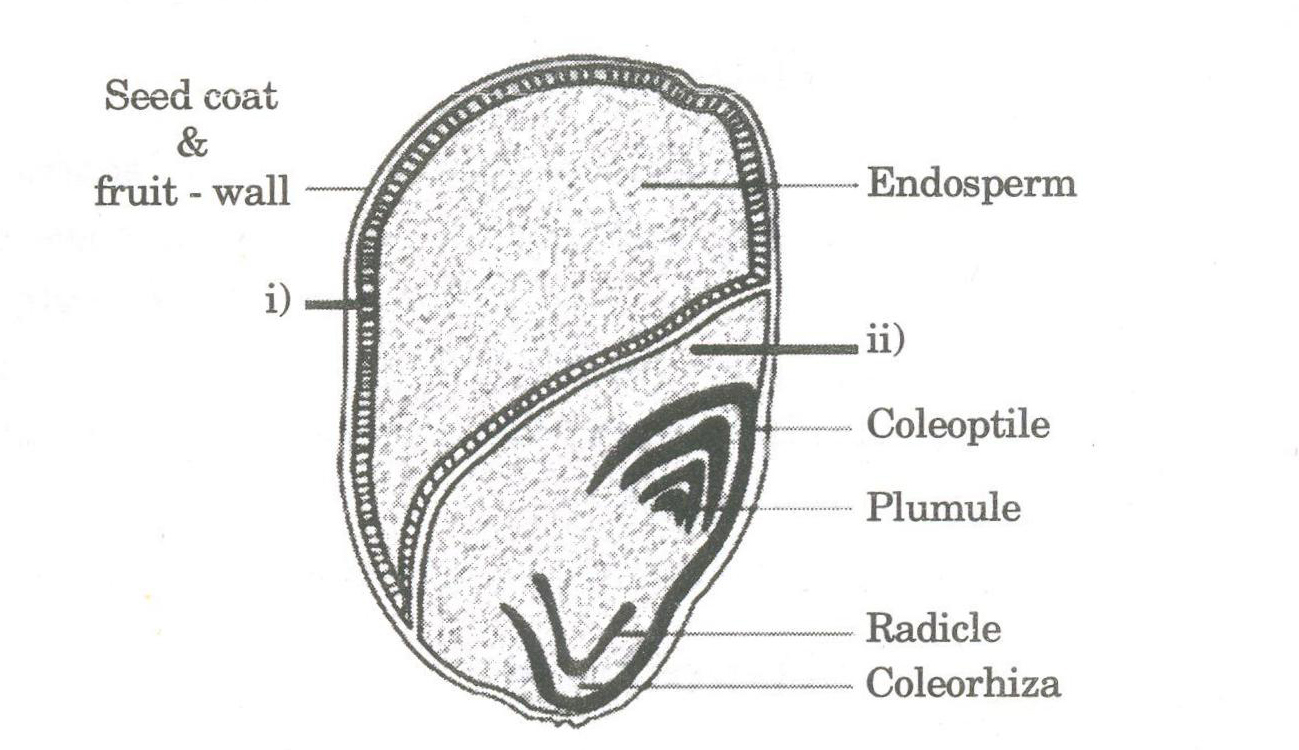The image is a detailed black-and-white diagram of a seed section, commonly found in science textbooks. Its oval shape is meticulously divided into various parts, each distinctly labeled. On the left side of the diagram, the outermost layers are marked as the Seed Coat and Fruit Wall. Towards the top of the diagram, the central area is labeled Endosperm. Descending down the diagram, the inner structures are sequentially labeled from top to bottom: Coleoptile, Plumule, Radicle, and Coleorhiza. This comprehensive labeling highlights the intricate layers and sections within the seed.